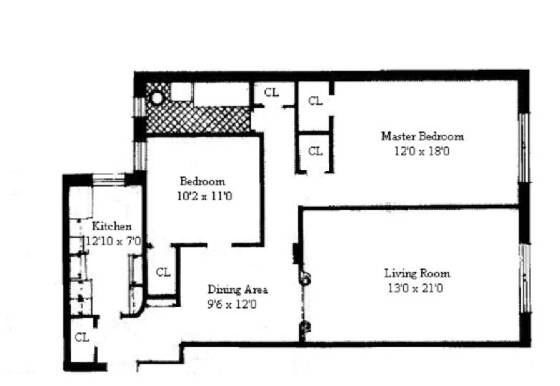This is a detailed floor plan of a residential space, possibly a house or an apartment, presented in a horizontal layout. 

### Upper Right Section:
- **Master Bedroom**: Positioned in the upper right corner, labeled with dimensions of 12'0" x 18'0" in black font. 
- **Living Room**: Located directly beneath the Master Bedroom, spanning 13'0" x 21'0". 
- A thick horizontal black line divides the Master Bedroom and Living Room, extending from the right edge to the center of the image.

### Right Edge:
- A very thick black line runs vertically along the right side of the image. 
- Two small white sections with black stripes are situated in the center of the right edge, one in the Master Bedroom and another in the Living Room.

### Upper Center:
- Two black rectangles labeled "CL" (closets) are positioned near the upper center, next to the Master Bedroom, separated by a vertical line. 
- An additional "CL" is located adjacent to these, maintaining continuity.

### Left Wall:
- **Bedroom**: Located on the left side, near the center, with dimensions of 10'2" x 11'0". The room is outlined in black and has an opening toward the right center for entry.
- **Dining Area**: Situated directly below this Bedroom, with dimensions of 9'6" x 12'0".
- An additional "CL" is found along the left wall, further down from the first Bedroom.

### Lower Section:
- **Kitchen**: Marked with dimensions of 12'10" x 7'0". It is positioned at the bottom and extends from the left to the middle. An opening at the bottom edge allows access.

The clear layout and detailed labeling suggest a carefully organized and functional living space, with distinct areas for sleeping, living, dining, and cooking.